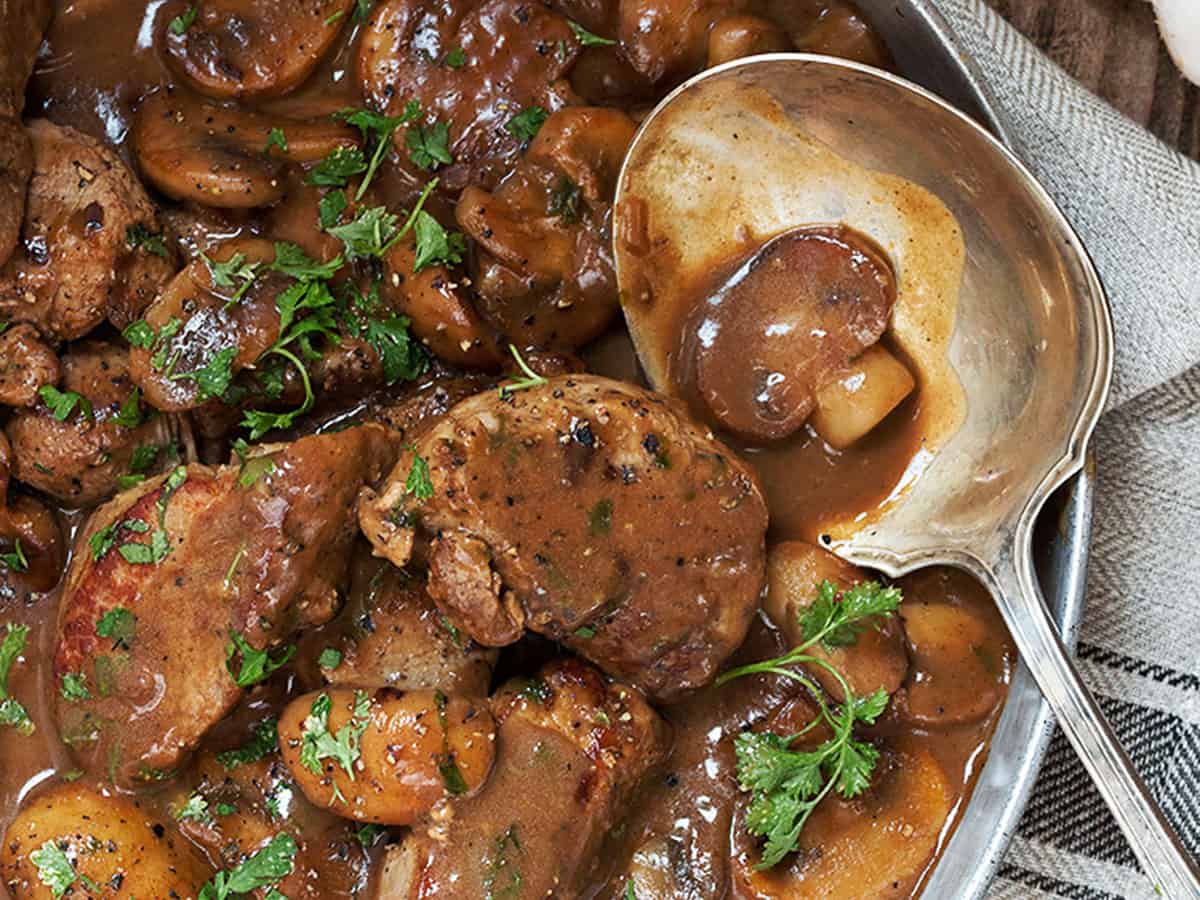This close-up photograph captures a mouthwatering serving of pork marsala with mushrooms. The meal is presented in a silver pan, possibly stainless steel, with various pieces of succulent pork and cuts of button mushrooms, all generously covered in a rich brown gravy. Sprinkled atop the dish are fresh green parsley leaves, adding a touch of color and freshness. A silver serving spoon rests on the edge of the pan, holding a mushroom slice drenched in the savory sauce. The pan is placed on a neatly woven napkin featuring light and dark gray stripes, which lies atop a dark wooden table partially visible in the upper right corner of the image. The entire scene is bathed in natural light, enhancing the delicious appeal of the dish.